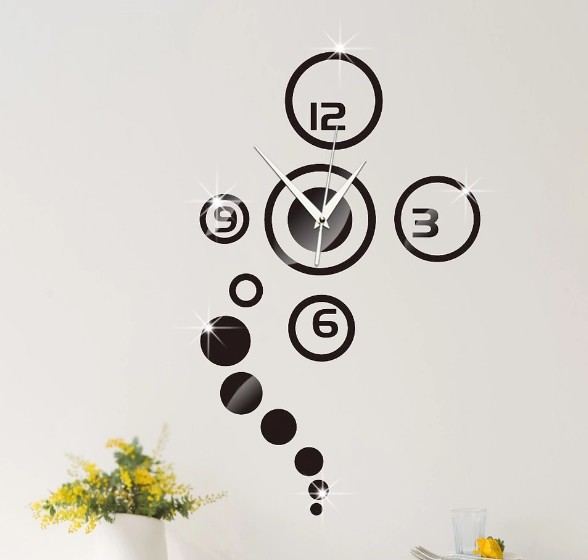This image features a minimalist and abstract clock design set against a white background with subtle decor elements. At the center is an abstract clock consisting of two overlapping circles: a smaller black circle within a larger white one, encircled by a thinner black ring. The clock face displays black numerals at the 12, 3, 6, and 9 positions, each encased in circles of varying sizes. The hour hand points to 1, the minute hand between 10 and 11, and the second hand extends straight up to 12. Radiating from these features are additional black circles of diminishing size, some of which sparkle like tiny stars, cascading towards the bottom left. Surrounding the clock, the bottom left corner showcases a small white flowerpot adorned with delicate yellow flowers and green leaves, while the bottom right corner houses a lone yellow flower and a cup, adding subtle life to the scene. The entire composition is set against a light grey wall, enhancing the striking simplicity of the overall layout.